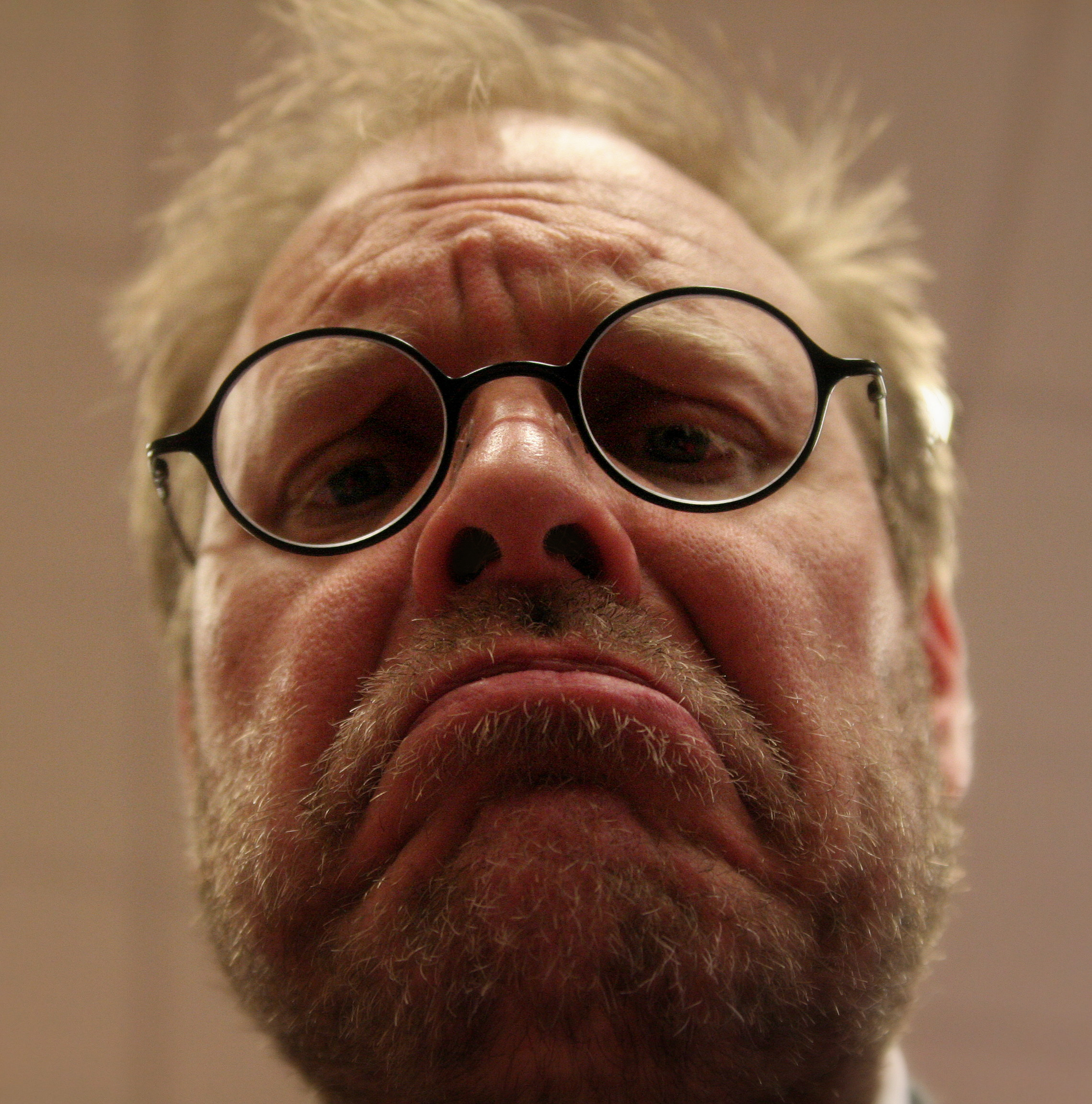In this detailed photograph, we see a close-up of a middle-aged man centrally framed, occupying most of the image. His short, possibly blonde hair contrasts with his dark brown eyes, which are behind round, black-rimmed glasses with clear lenses. His facial expression is characterized by an exaggerated frown, highlighting prominent frown lines and giving him an overall sad demeanor. The man’s facial hair is unkempt, featuring a scruffy beard and a mustache. The photo is tightly cropped, showing only his face from the lower chin upwards and omitting his neck. Behind him, the out-of-focus background recedes into a white drop-down panel ceiling and a white-painted wall, adding to the indeterminate indoor setting. The hues in the image include light brown, tan, gray, black, and pink, with the color of his clothing visible only at the bottom edge of the frame.